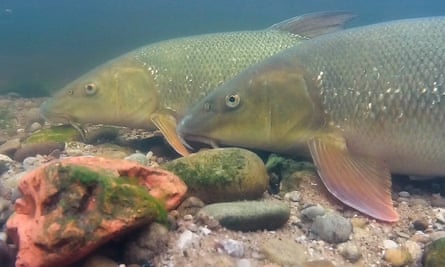Two bluish-gray fish with beady black eyes rest side by side at the sandy bottom of an aquatic setting, possibly a lake or ocean. Though unmoving, they appear to be at rest rather than deceased. Their side fins exhibit a distinctive purple-pink hue. The water is somewhat murky in the background, hinting at a not-too-deep location. The scene is adorned with rocks and pebbles, and an orange-colored shell or rock, overgrown with mossy green algae, adds a splash of color. The iridescent sheen on the fish’s gills and scales catches the light, creating a subtle glow. The foreground features another rock with a similar greenish growth, contributing to the overall textured and natural underwater landscape. The close-up nature of the image allows for clear enough visibility to appreciate the details of the fish and their surrounding environment.